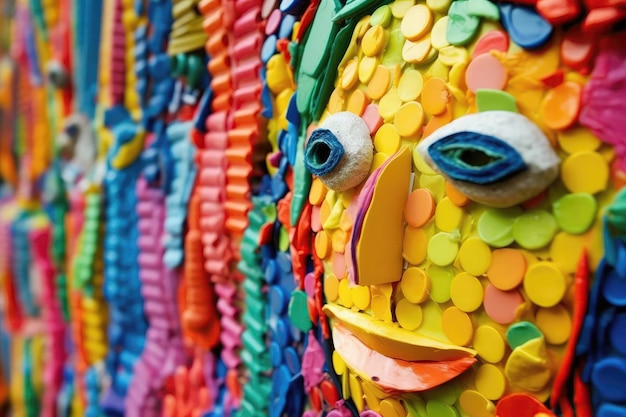This image captures a vividly decorated vertical surface, possibly a cake or a wall art, adorned with an array of bright, multi-colored elements that span the full spectrum of the rainbow. The scene is dominated by a highly detailed mask-like face positioned on the right-hand side. The face features oversized, expressive components, including large, doughy white eyes with blue ellipses that angle toward a protruding nose, which appears to be cut from yellow cardboard with purple edges. The mouth is composed of a pie-shaped upper lip and a striking orange lower lip. Surrounding the face are numerous round circles in yellow, green, pink, blue, and red. On the left side of the image, the surface is embellished with multicolored, wavy, tubular shapes that cascade out of focus, contributing to the overall sense of dynamic motion and vibrancy in this richly textured and colorful scene. The photograph captures this intricate decoration in a landscape orientation, highlighting the captivating blend of colors and textures in a style that borders on photographic representational realism.